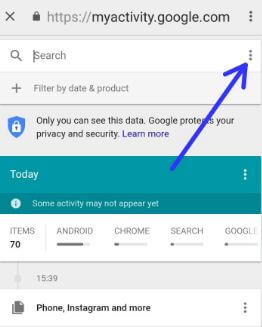Screenshot of the Google My Activity page. At the very top, there is a gray bar spanning the width of the screen, with the URL "myactivity.google.com" displayed prominently. On the far right of this bar, there is a vertical three-dot menu icon, while on the left, there is an X button for closing the window. Directly below the gray bar is a search bar aligned with another vertical three-dot menu icon on its right side, highlighted by a hand-drawn blue arrow pointing towards it.

Beneath this section, there is an option labeled "Filter by Date & Product" marked with a "+" symbol. Following this is a blue shield icon featuring a lock, accompanied by text that reads, "Only you can see this data. Google protects your privacy and security." A "Learn More" link is provided for additional information. Further down the page, a green bar displays the word "Today" on the left, alongside a vertical three-dot menu icon on the right. Below this, a message states, "Some activity may not appear yet."